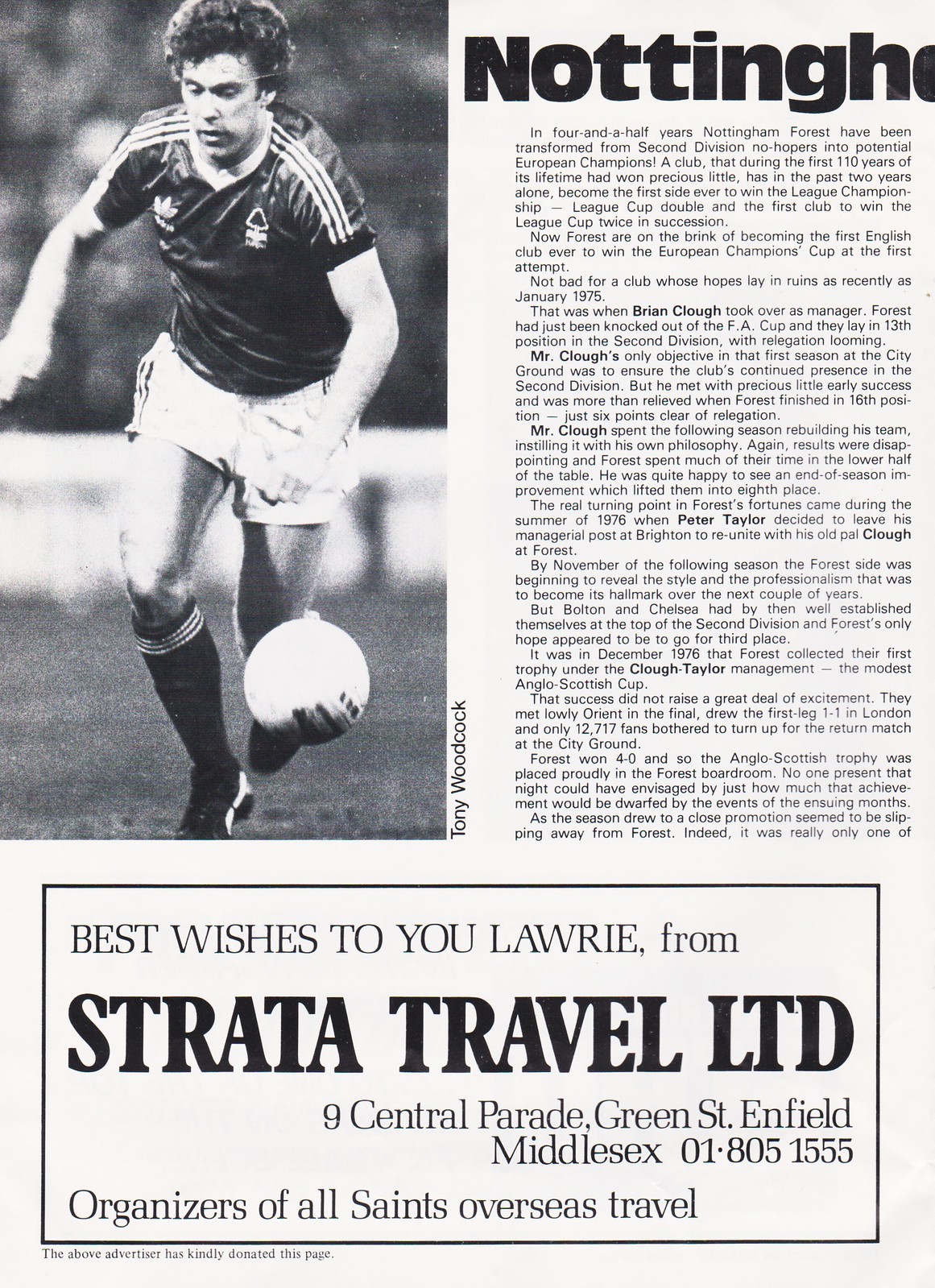The image features a black-and-white newspaper clipping with a large photograph of a soccer player—identified as Tony Woodcock—wearing a dark jersey, light-colored shorts, and dark socks. He is captured in mid-action, intensely running towards the ball. To the right of the photograph begins an article that discusses the remarkable transformation of Nottingham Forest under Brian Clough and Peter Taylor, including their achievements from near-relegation in January 1975 to potential European champions within four and a half years. The article details their rise, including winning the league championship, the league cup double, and their journey to possibly becoming the first English club to win the European Champions Cup in their first attempt. The clipping also includes a rectangular advertisement at the bottom, reading "Best wishes to Hugh Laurie from Strata Travel Limited, 9 Central Parade, Green Street, Enfield, Middlesex, 018051555." An additional note beneath the advertisement mentions that Strata Travel Limited has kindly donated the page.